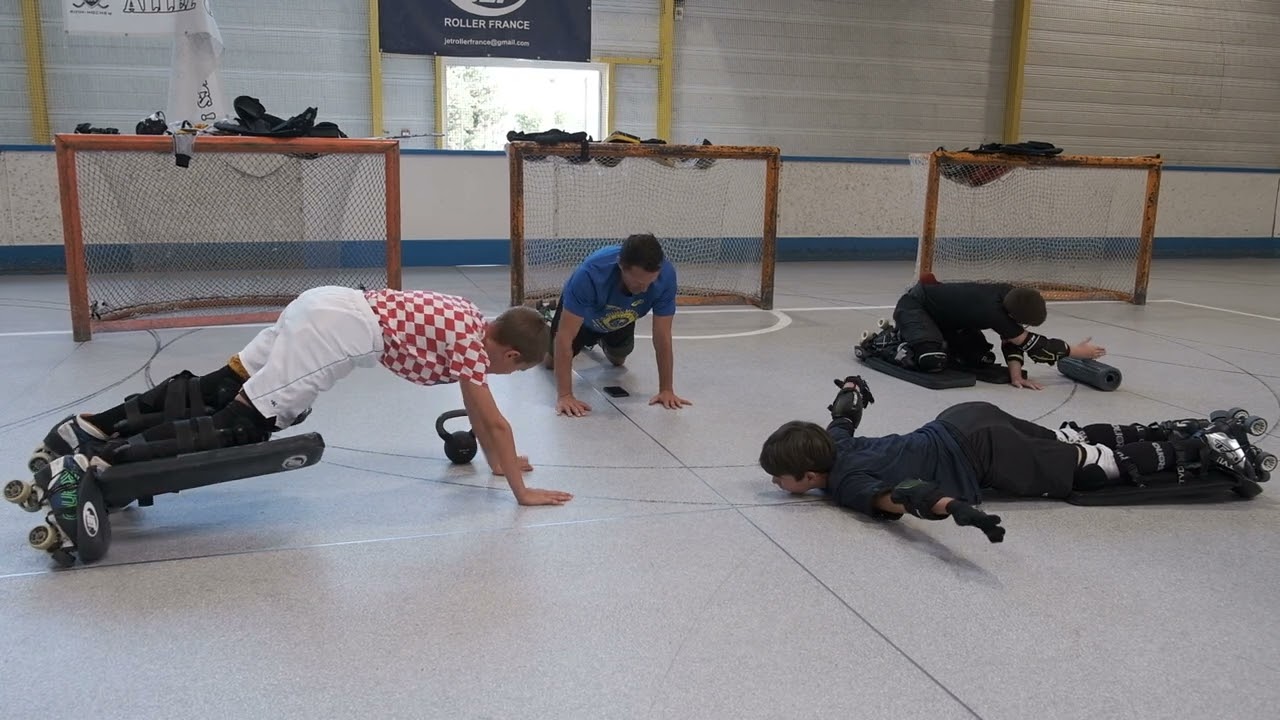This color photograph depicts a group of four individuals—three boys and one man—engaged in various exercises in the middle of a roller hockey rink. They are positioned in a circle, each performing different activities. All participants are equipped with roller skates featuring dark black knee pads that extend from the top of the skates up past their knees. 

On the left side of the circle, two people are doing push-ups. To the right, one person is lying on the floor with his hands positioned behind his back, while another is leaning toward the camera with his right arm extended over a foam roller, suggesting he is stretching. The man in the group is identifiable by his red and white checkered shirt.

In the background, there are three hockey nets with wooden frames and white netting. A sign that reads "Roller France" in white text against a blue background is mounted on the white corrugated wall. The entire scene is set in an indoor gymnasium, capturing the unique fusion of roller skating and physical exercise.